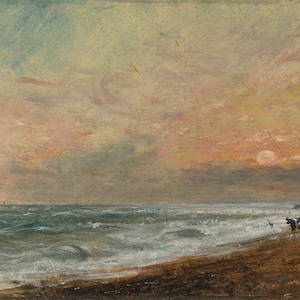A square fine art painting of a muted, dimly-colored beach scene captures the calm and desolate beauty of the shoreline at dawn. The bottom third of the painting features a grayish-blue ocean with choppy waves gently crashing onto a barren, dark sand beach. The shoreline traces a diagonal line from the lower left to the upper right, adding a dynamic element to the composition. An enigmatic black silhouette of an individual, faintly outlined, stands near the bottom right corner, gazing at the ocean. In the top two-thirds of the artwork, the sky unfolds in a palette of dark blues, grays, and hints of dark yellows, reds, and oranges, evoking a serene sunrise. The barely visible sun emerges from the vibrant center of the sky, adding a focal point to the tranquil scene. The mixture of muted hues creates a peaceful yet somber ambiance, making it a compelling piece suitable for display in a living room or office, inviting viewers to reflect on its serene beauty.